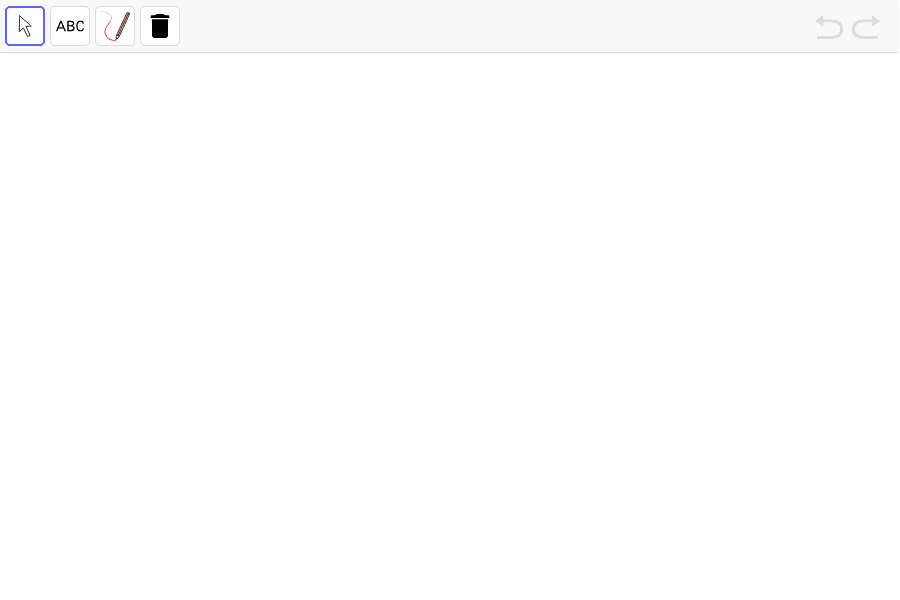This screenshot showcases a segment of an image editing software, specifically capturing a gray toolbar. On the left side of the toolbar, four square buttons are visibly aligned vertically. The first button displays a cursor icon and is highlighted in blue, indicating it is currently active. Next to it, the second button features the letters "ABC," followed by a third button adorned with a pencil sketching a red line, suggesting a drawing tool. The fourth and final button in this row presents a black trash can icon, likely a delete or remove function. On the far right of this toolbar, there are two additional controls: a back arrow and a forward arrow, both curved like the letter "C," presumably for undoing and redoing actions. The screenshot appears to have been cropped to focus entirely on this specific toolbar section, omitting the surrounding workspace and other interface elements.